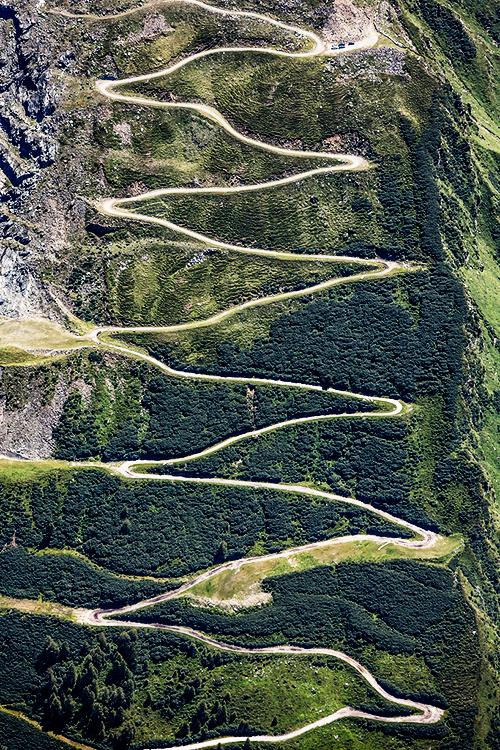This image captures a bright, daytime overhead view of a mountainous, countryside area rich with greenery and natural features. The aerial perspective highlights a winding road that zigzags through the terrain, resembling a series of V shapes or waves. This road, prominent and white against the verdant backdrop, traverses the mountainside, which is dotted with dark green patches of trees and scattered rocks. Towards the top left of the image, the mountainous region slopes downward to the right. Notably, there are three vehicles parked near the road's edge at the top of the image, suggesting a popular spot for hiking or camping. The overall scene blends rocky landscapes with lush vegetation, presenting a striking and detailed portrayal of the wilderness.